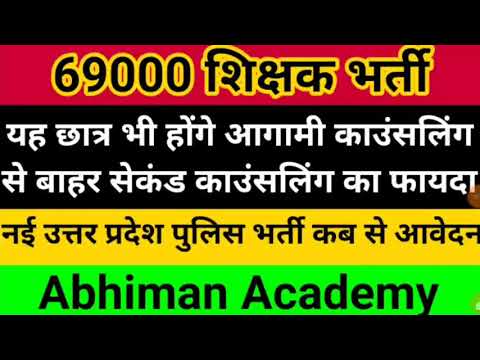The image appears to be a computer-generated advertisement with an intricate layout of colorful sections displaying predominantly foreign text, possibly in Arabic or an Indian language. At the very top, there is a solid black bar. Directly beneath it, a bright pink bar contains the bold text "69,000" in black and an underline in yellow, followed by two foreign words. Below this pink bar is a thicker black section filled with white foreign lettering; this black bar also includes a small orange icon on the lower right corner. Following this, there's a yellow bar adorned with additional foreign text in black font. At the bottom is a green bar displaying "Abhimanyu Academy" in black lettering. The alternating black and colored sections, combined with diverse fonts and languages, suggest this could be an advertisement for a school or educational institution, with details possibly about fees or services.